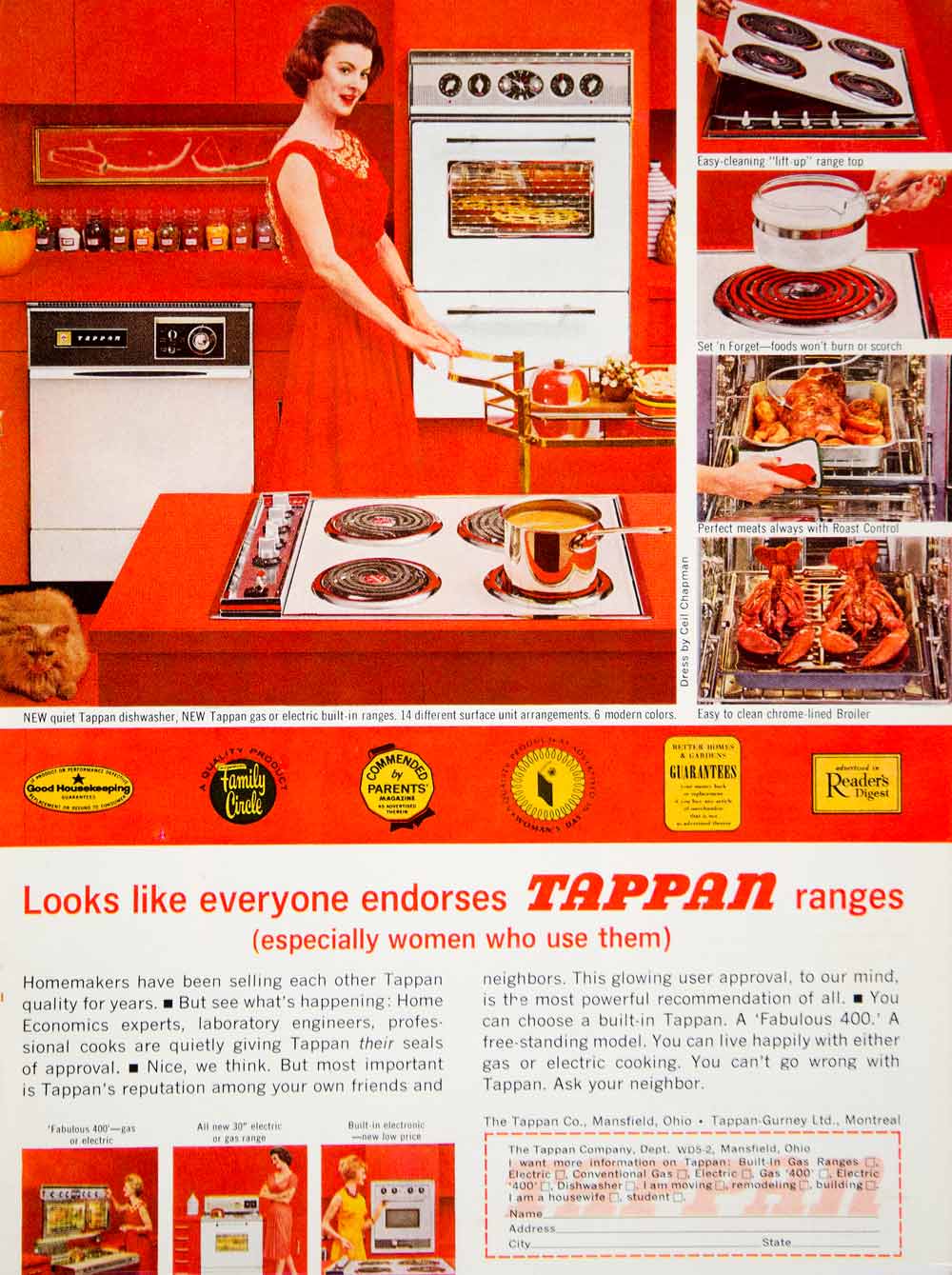A nostalgic 1960s newspaper clipping showcases a vibrant red kitchen where a housewife in a red dress is pushing a golden serving cart laden with food. Behind her, a sleek, chrome-lined built-in oven is spotted with what might be a baking pie, while to her right stands a white dishwasher, with a shelf of spice canisters above it. The heart of the image is dominated by a striking red, four-burner stovetop with one burner glowing red beneath a pot filled with an orange substance. Also catching the eye is an orange tabby cat lounging on the floor.

Details at the bottom of the image highlight the new Tappan appliances: a quiet, tap-on dishwasher, and a tap-on gas or electric built-in range with 14 different surface unit arrangements, offered in six modern colors. A series of four smaller images to the right illustrate various functionalities: lifting the stovetop burner for cleaning, a pot on a glowing coil, a chicken being roasted, and two lobsters in the oven.

Red text declares, "Looks like everyone endorses Tappan ranges, especially women who use them." Further text underscores Tappan's wide endorsement from homemakers to professional cooks with exemplary user approval. Additional small images at the bottom left show women utilizing each appliance—a dishwasher, an oven, and a stovetop range. There's a call to action to inquire more about Tappan products, providing a clip-out coupon for potential customers to request information, emphasizing Tappan's trusted reputation.